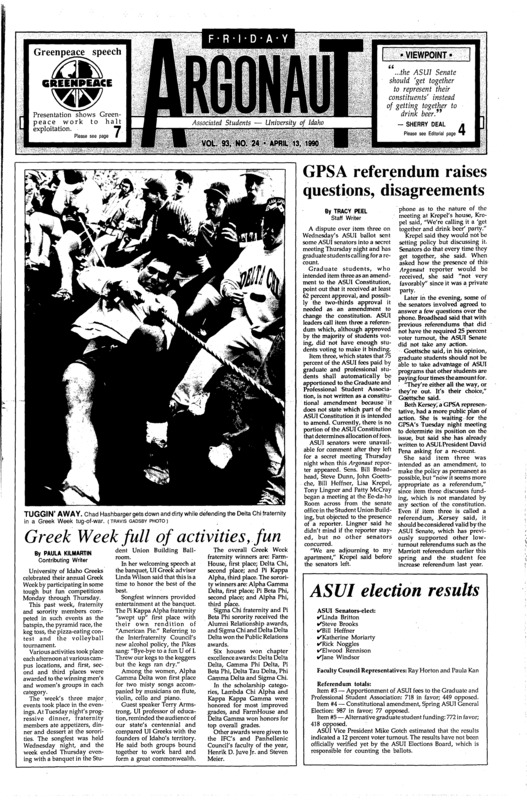The image is a low-quality, black-and-white scan of the front page of the University of Idaho's college newspaper, the Argonaut, dated April 13, 1990. The masthead reads "Friday Argonaut" with "Friday" accented by dots between each letter in a black rectangle background. This edition is Volume 93, Number 24. Prominently featured is the headline "Greek week full of activities, fun" accompanied by a photo showing students engaged in a tug-of-war, likely between fraternities. Above this central image is an advertisement for a Greenpeace speech. Another major headline reads "GPSA referendum raises questions, disagreements," with a detailed article below. The lower right-hand corner of the page includes a box labeled "ASUI election results" with associated details. The newspaper is scanned in grayscale, emphasizing its archival nature.